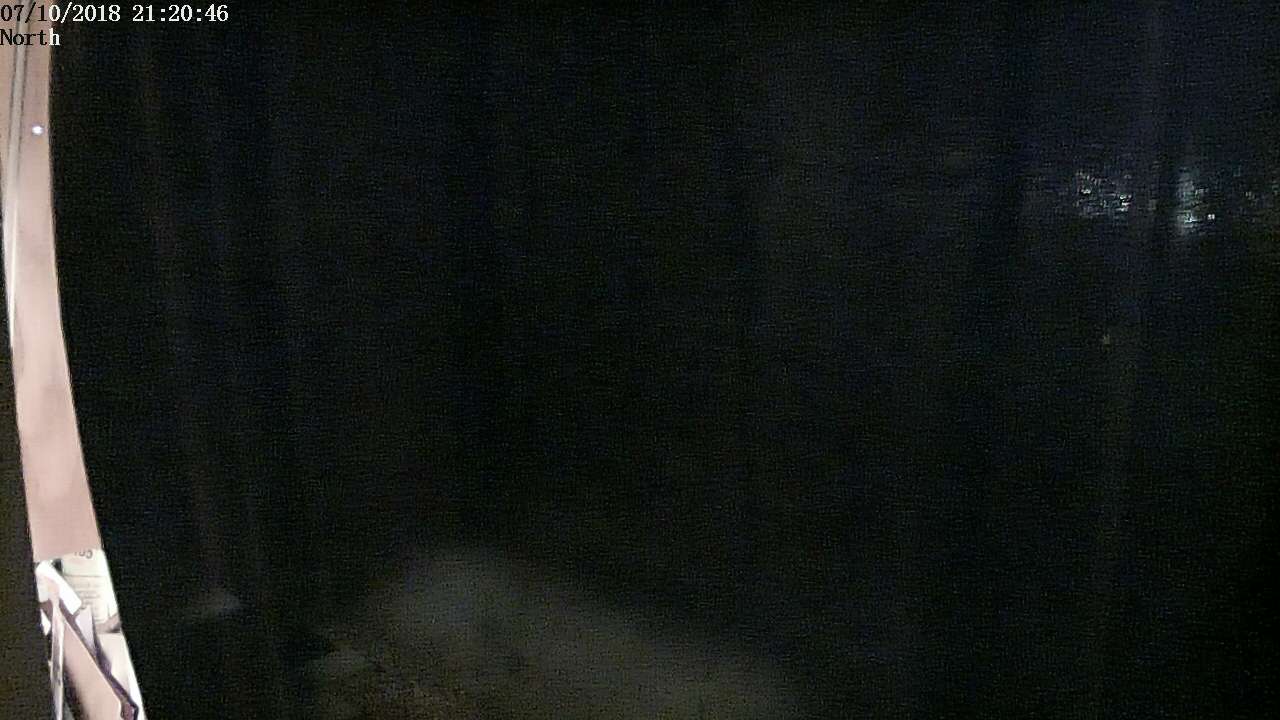This photograph, captured by a security camera, appears to be taken from a yard during nighttime. Dominating the image is an expanse of darkness, emphasizing the lack of illumination in the environment. To the left, a gray section introduces a slight contrast, but the ambiguity of this area makes it difficult to discern whether it is a doorway, a garage opening, or another feature. In the top left corner, a timestamp dated 7-10-2018 at 21:20:46 is visible, along with the directional label "North." On the right side, the pitch-black scene is interrupted by splotches of white, possibly indicating a distant light source, although the details remain indistinguishable due to the poor lighting conditions in the photograph.